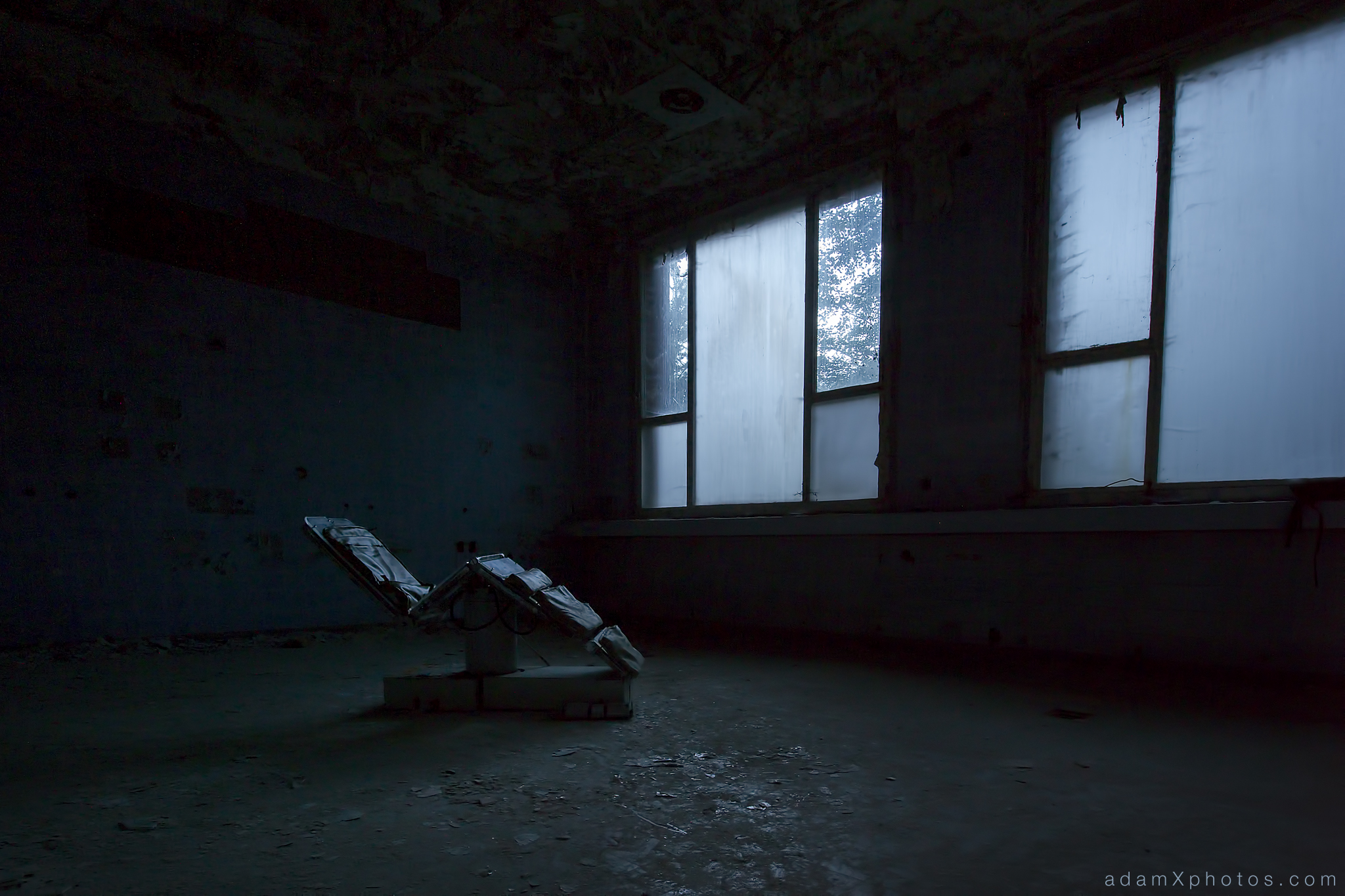In the eerie photograph taken inside an abandoned building, the scene is meticulously captured in a bluish-gray monotone. The ceiling has deteriorated, with mold evident, adding to the somber ambiance. The cinder block walls display peeling paint, while the concrete floor reinforces the cold, desolate atmosphere. Two large windows, mostly opaque, allow only a trickle of natural light to filter through a couple of clear panes, casting minimal illumination and contributing to the sense of isolation. Central to the room is a dental chair, reminiscent of an ominous torture device, its presence intensified by the darkness. The remnants of a ceiling light fixture hint at the building's dilapidated past. In the lower right corner of the image, "adamxphotos.com" marks the photographer's signature, solidifying the haunting mood of this forsaken, possibly wintery, location.